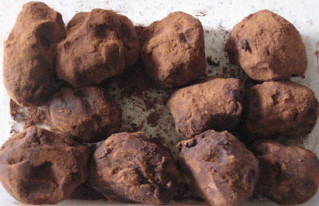This digital photograph showcases an arrangement of 11 brown clay-like balls on a white surface, organized in three rows: four balls on the top row, three in the middle, and four on the bottom. The balls are not perfectly spherical, exhibiting a round yet varied shape with some oval and oblong forms. Their surface appears lumpy and features various shades of brown, with the top row displaying a lighter hue compared to the darker balls at the bottom. The texture of these clay or dirt-like objects is crumbly, with some having noticeable dents and a chunk missing from the one in the lower left corner. Scattered around the balls is a light brown powdery substance, possibly residue from the balls themselves, adding to the overall gritty and earthy appearance of the scene.